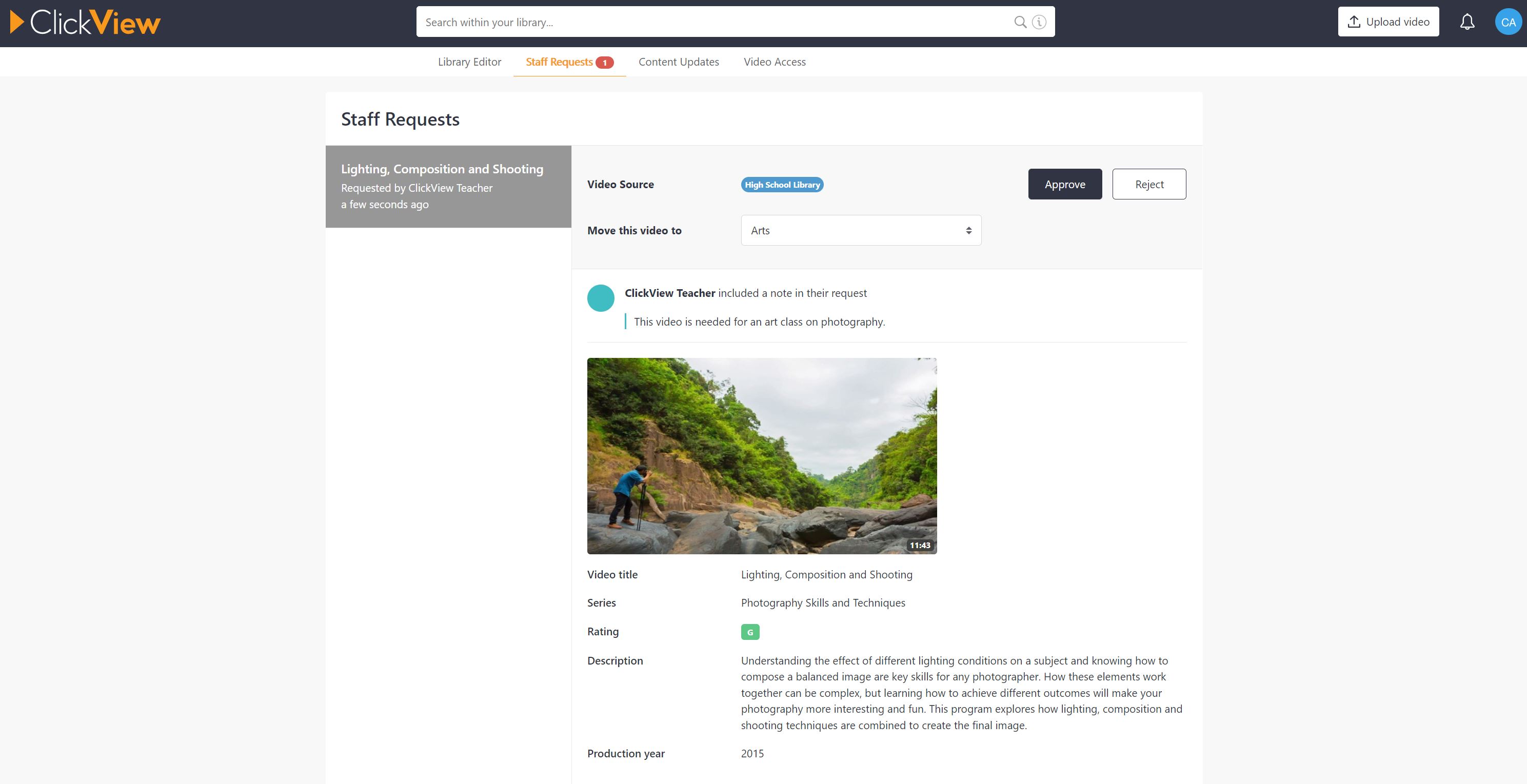Screenshot of ClickView Website Interface

The screenshot captures the ClickView website interface. Prominently displayed is a yellow triangle icon pointing to the right, symbolizing a play button. The brand name "ClickView" is presented with "Click" in non-bold, white lettering and "View" in bold, orange lettering, distinguishing the two parts of the name effectively.

Centered at the top, there is a search bar with the placeholder text "Search within your library," allowing users to easily locate content. Adjacent to this, in the top-right corner, are an upload button, a notification bell icon, and user info.

Directly below the search bar, a four-button menu provides quick navigation options: Library Editor, Staff Requests, Content Updates, and Your Access/View Access. 

The highlighted section of the page is "Staff Requests," indicated by the header on the left-hand side. Under this header, there are options including "Video Source" and a blue circle icon with the label "High Speed Choice." Below this, there are controls such as "Make this video" and "Move this video to," accompanied by a dropdown menu for further selections.

A detailed portion of the interface includes a screenshot of the video in question, alongside its title, rating, and a brief description, providing essential information at a glance.